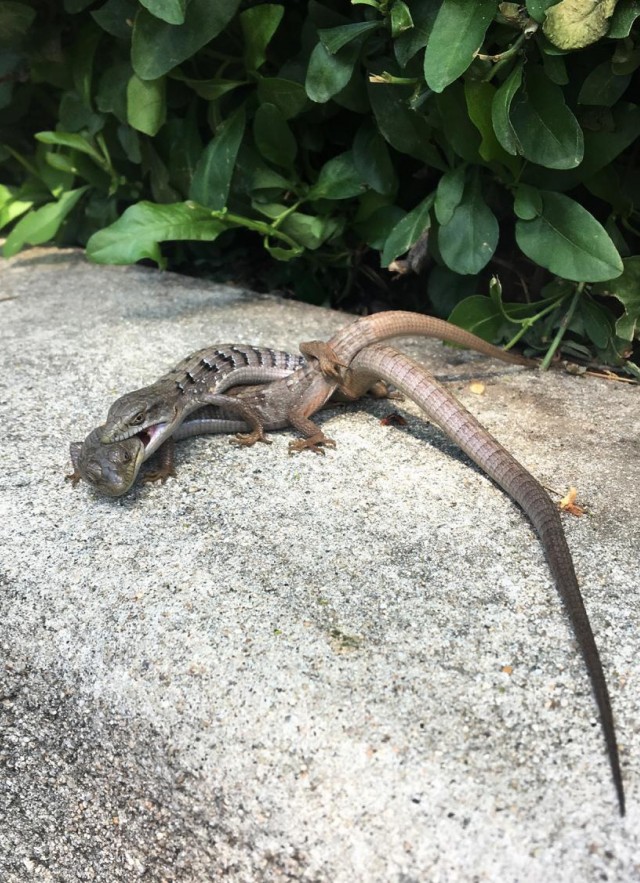This vertically oriented photograph captures a dramatic and surreal moment in nature, where a snake and a lizard are engaged in a fierce battle atop a large, multicolored granite rock, set amidst lush green foliage. The snake, detailed with prominent black stripes along its back, is poised on top of the browner lizard, aggressively sinking its fangs into the lizard’s head. The lizard, seemingly lifeless with closed eyes, has a notably long tail that trails off to the right, nearly reaching the bottom corner of the image. The rock underneath them has distinct white, brown, and black sediments, contrasting with the vivid greenery in the background. This intense struggle atop the rock unfolds against a backdrop that suggests a natural, jungle-like or woodland setting.